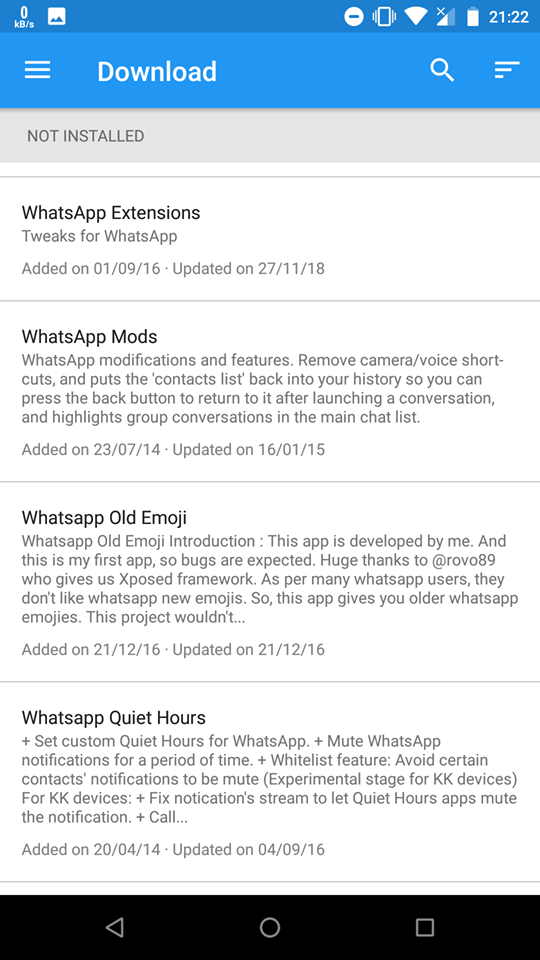Screenshot of an Android Phone Displaying Download Information

In this screenshot of an Android phone, various interface elements and app details are prominently featured. In the upper left-hand corner, "0 KB/s" is visible, accompanied by a small mountain icon. The upper right-hand corner shows the time as "21:22" in military time and indicates a battery level around 80%. The phone is set to vibrate mode.

The main screen title reads "Download." In the top left corner, a menu icon comprised of three horizontal white lines is displayed. On the right side, there’s a magnifying glass symbol for search functionality, followed by another menu icon with three horizontal lines of varying lengths.

Below the title "Download," it states "NOT INSTALLED" in capital letters. The following details about various WhatsApp-related tweaks and extensions are listed:

1. **WhatsApp Extensions**:
   - **Description**: Tweaks for WhatsApp
   - **Added On**: 01/09/16
   - **Updated On**: 27/11/18

2. **WhatsApp's Mod**:
   - **Added On**: 23/07/14
   - **Updated On**: 16/01/15

3. **WhatsApp Old Emoji**:
   - **Added On**: 21/12/16
   - **Updated On**: 21/12/16

4. **WhatsApp Quiet Hours**:
   - **Added On**: 20/04/14
   - **Updated On**: 04/09/16

The layout of the information is clear, making it easy for the user to understand the status and details of various WhatsApp modifications.